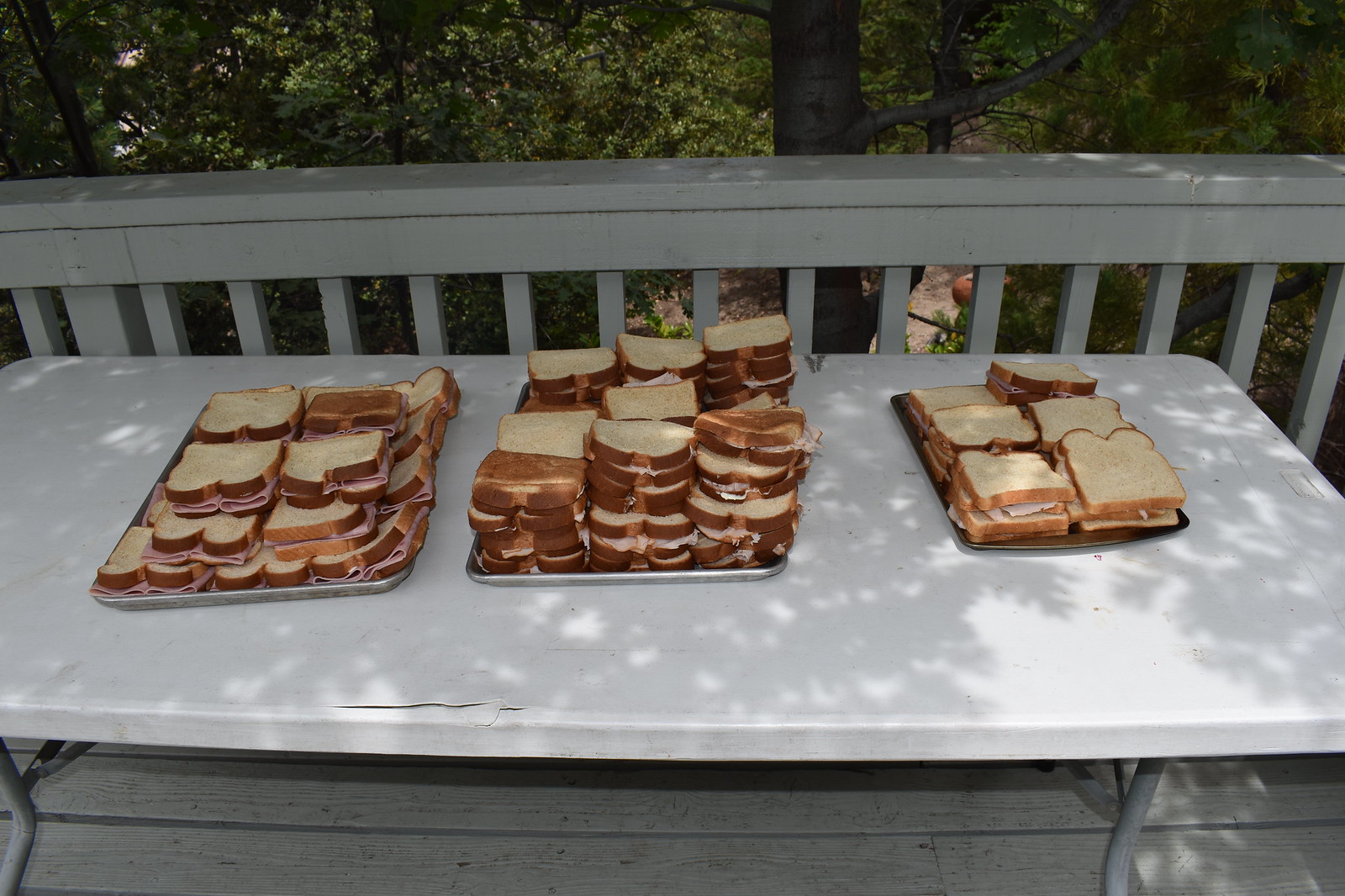The image depicts a white plastic folding table with silver metal legs, situated on a gray-painted wooden deck or porch, with gray railings featuring vertical pillars behind it. A lush backdrop of green trees and vegetation is visible beyond the railing. On the table are three trays of sandwiches: the left and middle trays are larger and made of metal, while the right tray is slightly smaller and possibly brown. The middle tray holds the most sandwiches, appearing to be stacked four high, and the right tray has the least, stacked two high. The sandwiches feature light brown bread with crusts, containing various fillings; the left tray appears to have ham sandwiches, the middle tray's filling is indistinct, and the right tray likely contains turkey or chicken sandwiches. Sunlight casts shadows across the table, adding to the outdoor picnic ambiance. Additionally, a cylindrical pot can be observed on the ground between the trees in the background.